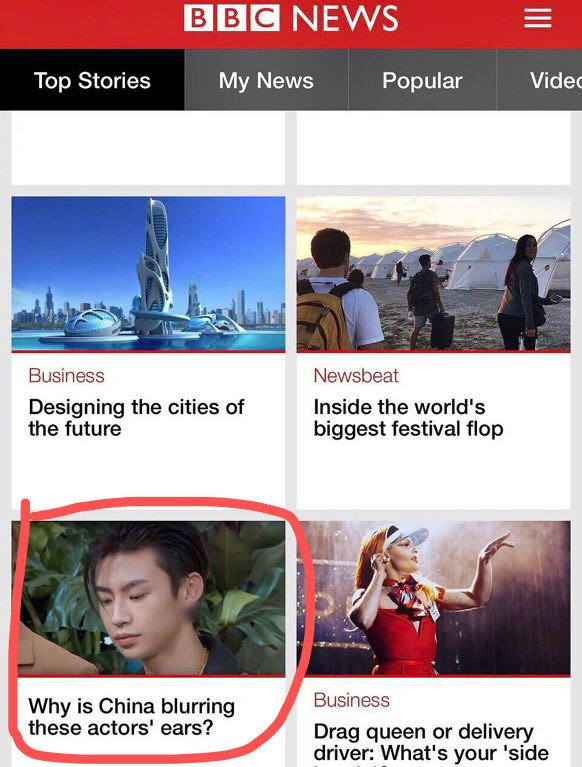This is a screen capture from the BBC News homepage. At the top of the screen is the BBC News logo accompanied by four navigation tabs: Top Stories, My News, Popular, and Video. The 'Top Stories' tab is currently selected. Below this navigation bar, four news stories are displayed:

1. **Business: Designing the Cities of the Future** - The accompanying image is a high-tech, futuristic illustration of a skyscraper.
   
2. **Newsbeat: Inside the World's Biggest Festival Plop** - The image shows four individuals standing in a desert-like area, seemingly part of a camping setup.

3. **Why is China Blurring These Actors' Ears?** - This headline is circled in red and features an image of a presumed Chinese actor with stringy black hair.

4. **Business: Drag Queen or Delivery Driver? What's Your Side?** - The headline is truncated and unclear beyond "Side." The accompanying image shows a woman performing on stage, wearing a cap and red dress.

The concise layout and vivid images draw the reader into the current top stories, emphasizing varied topics ranging from futuristic urban design to cultural phenomena in China.